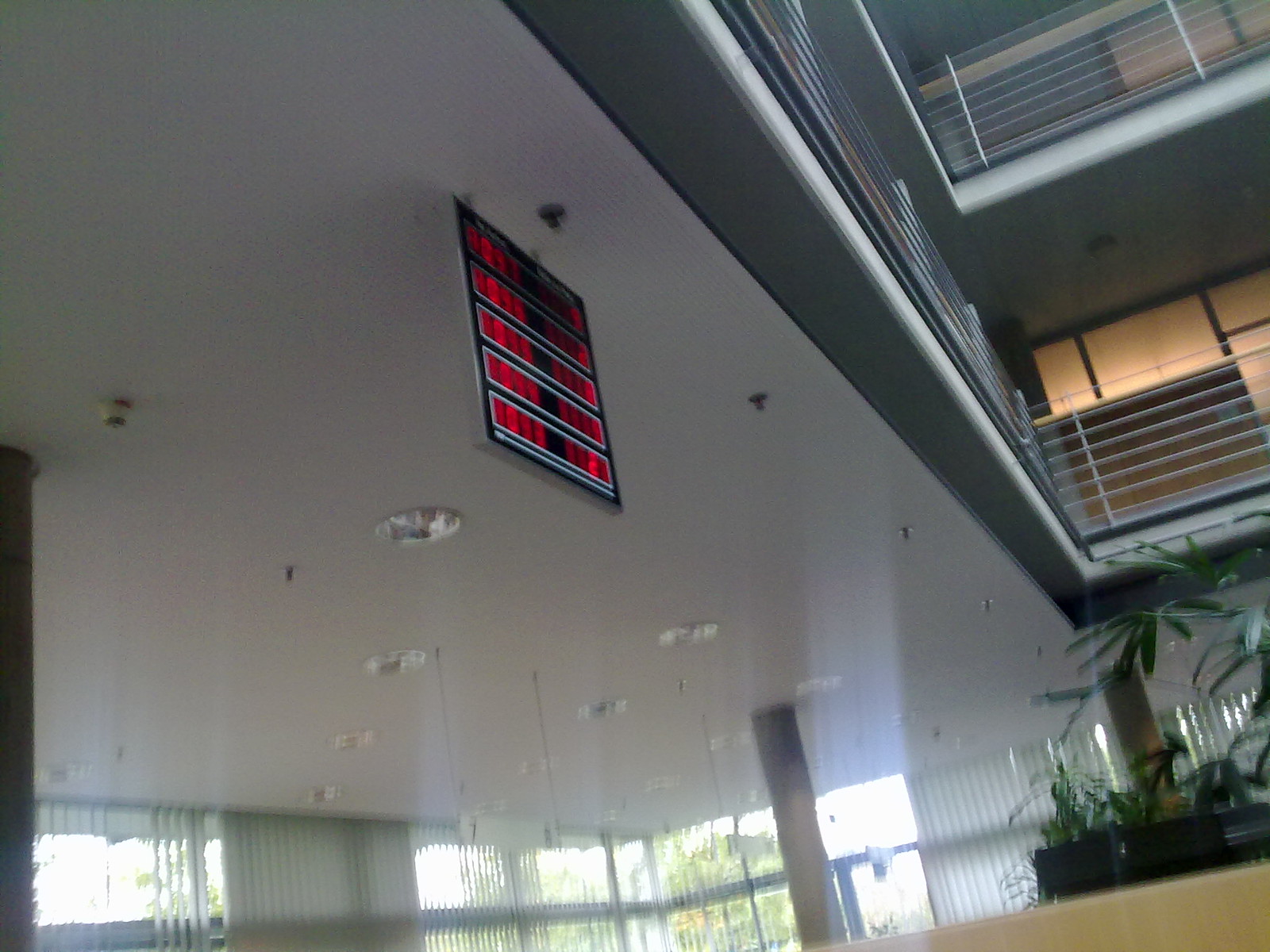The image depicts an indoor scene that appears to be a multi-level commercial structure, possibly a DMV, office building, hotel, or transportation hub like a train or bus station. The first floor has high, elevated ceilings equipped with circular canister lights, security cameras, and sprinkler heads. A prominent digital sign with red lettering displaying alphanumeric codes such as "A-22," "B-64," and "C-3" hangs from the ceiling, reminiscent of signage used for calling out numbers in queue systems at DMVs or other service areas.

Surrounding the central open area on the first floor are floor-to-ceiling windows adorned with vision blinds. The space also features potted plants, lending it a lobby-like atmosphere. The architectural layout includes visible railings leading up to balconies of the second and third floors, suggesting either additional business offices or apartments. The overall image quality is slightly blurry, with some portions out of focus, particularly affecting the clarity of the digital sign which also displays "1053" among other numbers. This multi-story space combines elements of functionality and aesthetic greenery, underlined by a sense of security and structured organization.